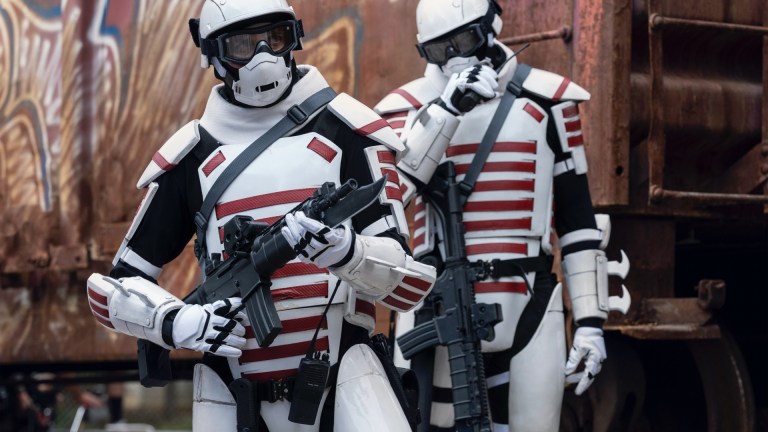The image depicts two robotic figures, resembling characters out of a science fiction universe, dressed in white armor with distinctive features. They wear white helmets paired with black goggles and white face masks, giving them a futuristic, militaristic appearance. Their armor includes a black underlayer, with white, hard plastic covering their chest, shoulders, forearms, thighs, and legs. The chest plates and shoulder pads are marked with red horizontal stripes, while their forearms are covered with glove-like armor that extends to the elbows. Each figure holds a black weapon resembling an assault rifle, complete with a knife blade attached near the muzzle. They are positioned in front of a rusty metal structure, possibly a building or train cart, with graffiti in various shades of brown and purple visible in the background. One of the figures appears to be interacting with a communication device, possibly a walkie-talkie.